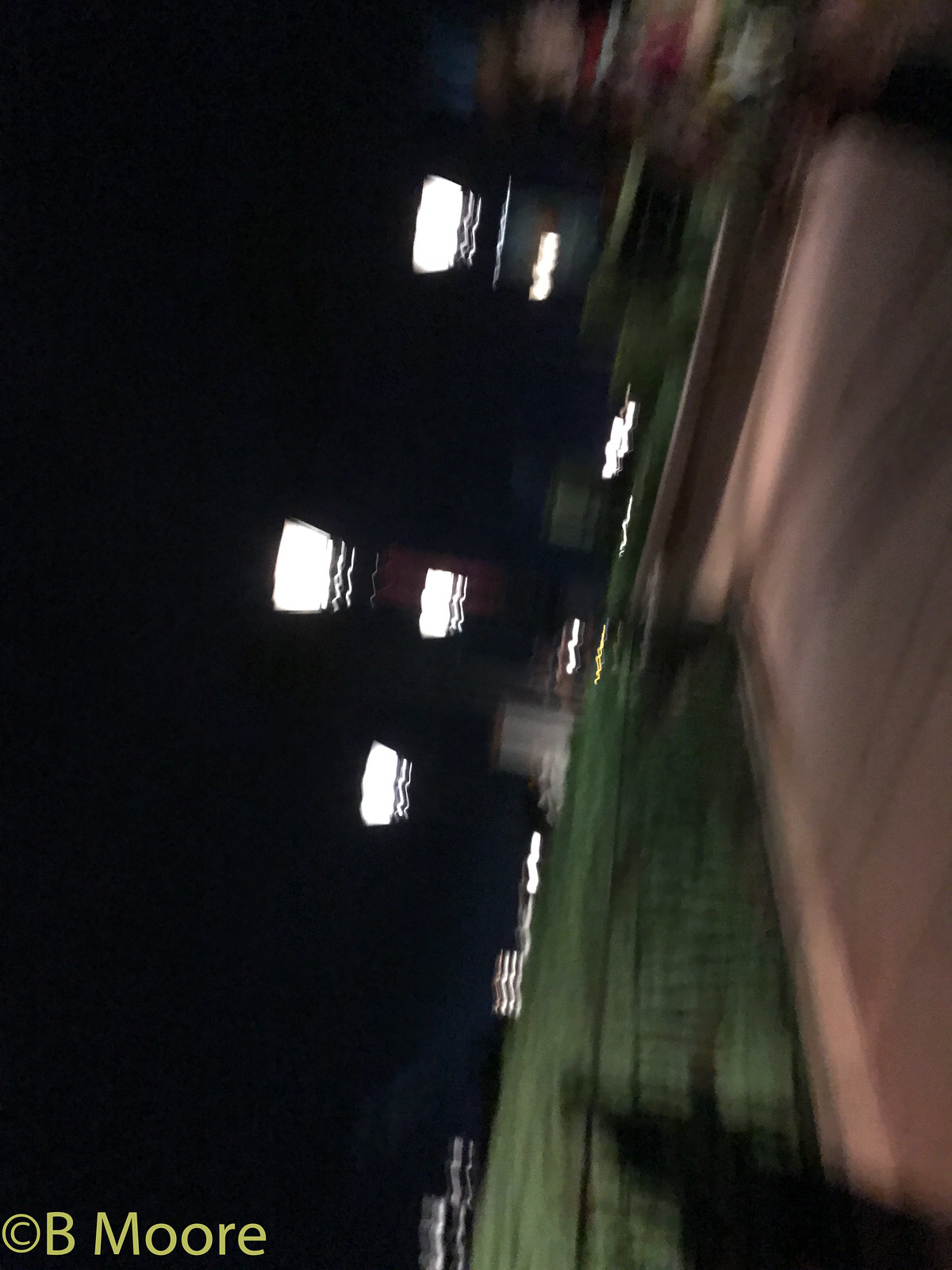This blurred, nighttime photograph was taken vertically and is slightly tilted to the right. In the foreground, there is a greyish or beige concrete driveway leading to the street, accompanied by shadows and light glares scattered throughout the image. The left side features greenery, likely a lawn, partially obscured by what seems to be a fence or its shadow. There are several illuminated streetlights visible, contributing to the overall blur and light glare in the scene. In the background, blurred buildings with bright white lights can be faintly seen against the pitch-black sky. Multiple colors—reds and greens—appear towards the top right of the image, possibly indicating a person walking out of the frame. The bottom of the picture bears a yellow copyright notice reading "B Moore," suggesting the photographer or the entity responsible for the image.